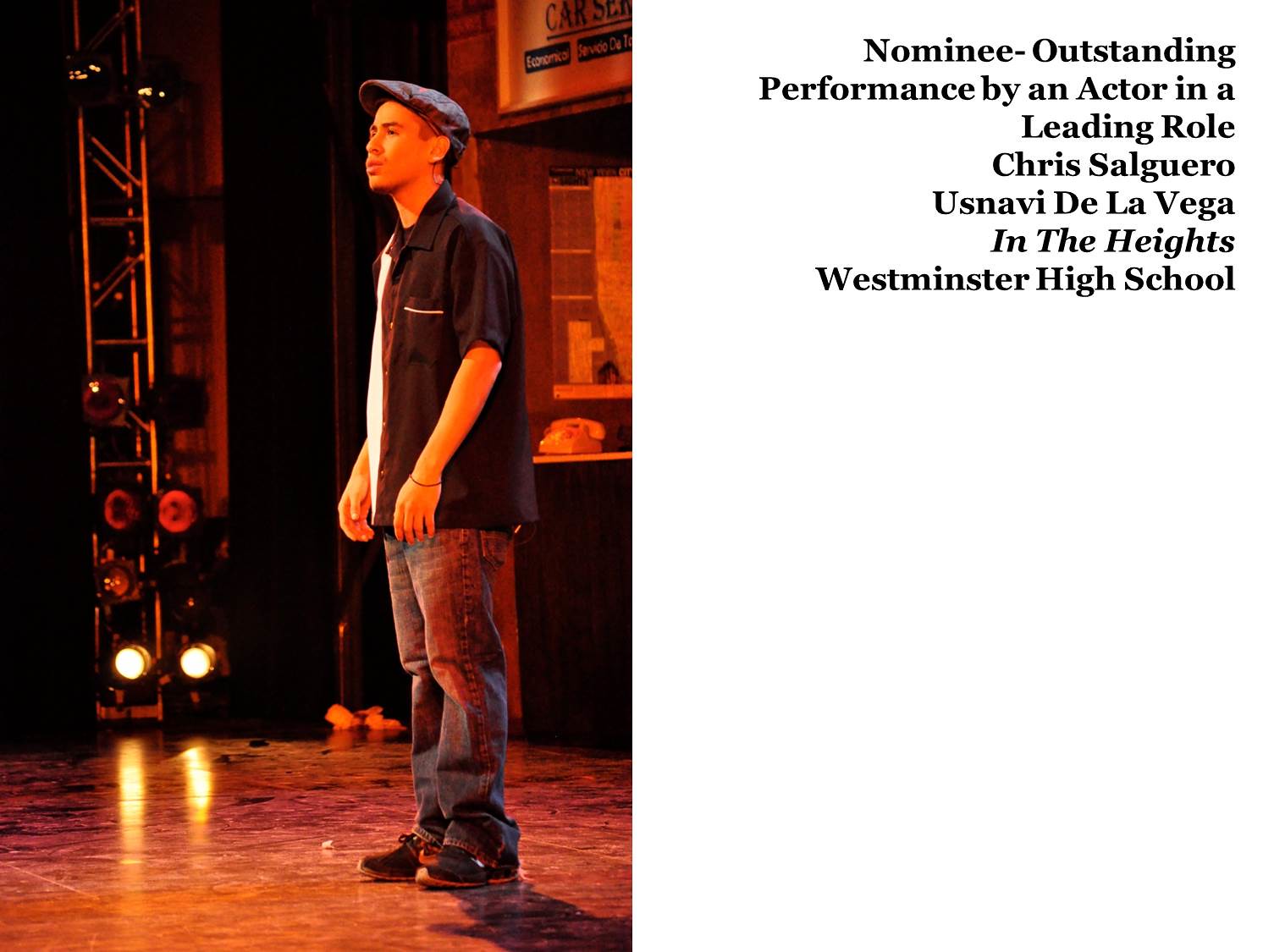The image features a young man, likely in his late teens or early twenties, captured in a dynamic moment on stage during a theatrical performance. Identified as Chris Talguero, portraying the character Usnavi de la Vega in "In the Heights" at Westminster High School, he is dressed in dark jeans, a white button-up shirt, a black jacket, brown shoes, and a distinctive cap that could be a bowler's cap. Stage lights illuminate him, highlighting his focused expression as he engages with the audience, reinforcing the dramatic atmosphere. Behind him, elements of the set such as a telephone, signs, and possibly maps are visible, enhancing the stage's realism. To the right of the image, a text overlay states his nomination for the Outstanding Performance by an Actor in a Leading Role, celebrating his contribution to high school theater.